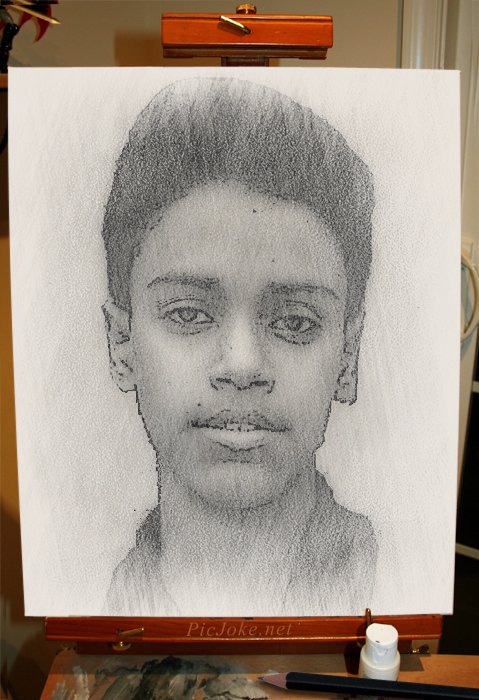The image depicts a digitally edited photograph designed to resemble a hand-drawn picture, though it clearly does not achieve this effect. The primary focus is a large white canvas mounted on a stand, prominently marked with "pickjoke.com" at the base, indicating the website that created the digital rendition. Although intended to mimic a sketched appearance, the canvas instead displays a black and white photo that has merely been passed through a filter. Below the canvas stand, a piece of cardboard smeared with dried paint suggests an attempt to evoke an artistic environment. Nearby are scattered tools of the trade: a black pencil and an indistinct white bottle, possibly holding some kind of art supply. The overall composition suggests an artificial effort to create an artistic scene, but the obviously filtered photo and contrived setup undermine the intended authenticity.